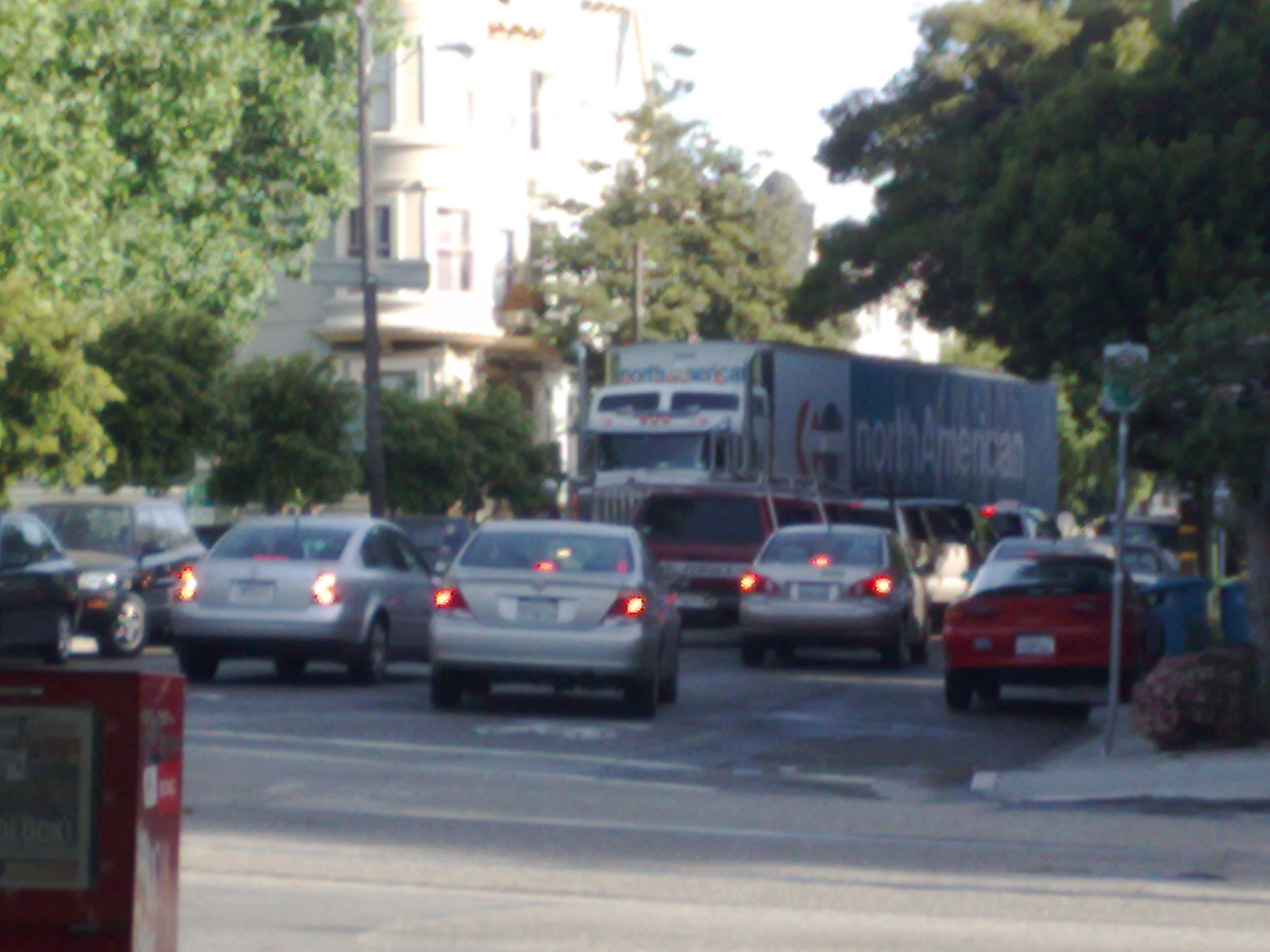The photograph captures a bustling urban street scene, likely situated in America, showcasing a busy junction with several cars queued up behind each other, potentially due to a red light. On the right side of the street, multiple cars are stopped, including a prominent red Honda. Both sides of the street are lined with trees, framing the image and adding a touch of greenery to the cityscape.

In the foreground, a red object, possibly a fire hydrant or newspaper dispenser, is visible. The street is divided into multiple lanes; on the right, three lanes of traffic head towards the foreground of the picture, and there's a lane of traffic going in the opposite direction. Among the vehicles, a significant number of silver cars have their brake lights on, suggesting they are at a standstill. 

In the distance, a large semi-truck with "North America" written on its side in white lettering against a light blue background can be seen navigating the road. Overhead, a modern, contemporary tan building with rounded corners and numerous windows looms high, adding to the urban atmosphere. Additional details include parked cars along the sidewalk, a bush, and a parking sign on the corner, with some telegraph poles standing further in the background under a partially cloudy, light sky.